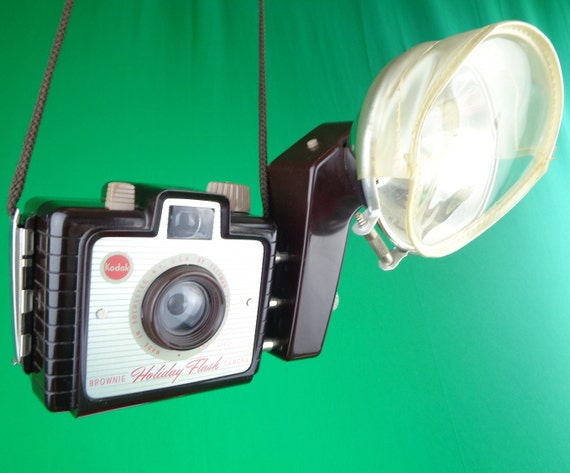The image displays a close-up view of a vintage Kodak camera set against a slightly bunched up, greenish fabric background. The camera, suspended by a small piece of rope, features a predominantly black body with a white front panel. Prominently displayed to the left side of the camera is a red label with white lettering, reading "Kodak," which is situated on a circular red background. The camera model, "Holiday Flash," is inscribed below the circular lens at the front center. On the right side of the camera, there's a large, black flash attachment enhancing the nostalgic feel of the scene. The image is bright and well-lit, emphasizing the camera's intricate details, including a viewfinder directly above the lens and a couple of control buttons on its upper section.